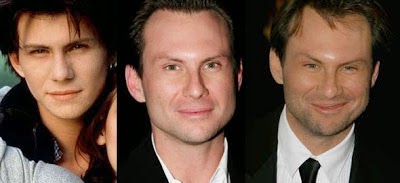The image displays a triptych of headshots featuring actor Christian Slater, showcasing his transition over the years. The composite measures approximately three inches wide and one inch tall, with each individual photograph being about an inch square. 

In the left photograph, a young Christian Slater, likely in his late teens or early twenties, is captured looking directly at the camera. His hairstyle is longer and touches his ears, and he wears a gray top with a black collar. This image appears to be from one of his early movies, as indicated by the partial face of a young woman in the lower right corner, over whose shoulder Slater is peering.

The middle photograph presents a more mature Slater, possibly in his mid-30s. His hair is slicked back, signaling a shift from his earlier style. He wears a black jacket over a white shirt, with his facial features appearing more squared and defined.

The right photograph depicts Slater at a similar age to the middle photo, but with a more relaxed demeanor. His hair is messier, and he sports a broad smile. He is dressed in a black dress jacket, a white button-up collared shirt, and a black tie.

Together, the images chronicle the actor's visual transformation over time, portraying changes in his hairstyle, attire, and overall demeanor.